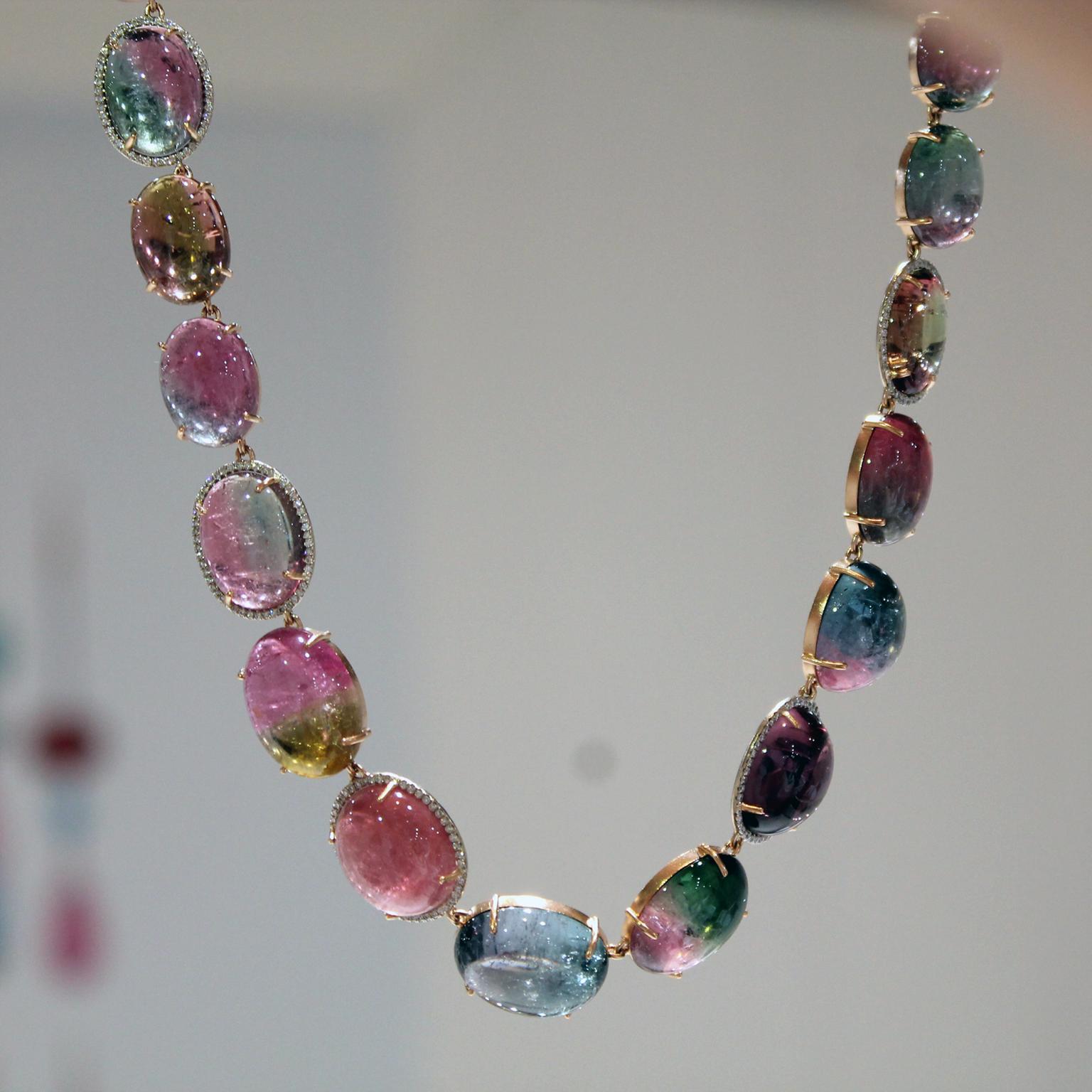This image features an exquisite necklace gracefully hanging against a light gray background that appears blurred. The necklace showcases an array of vividly colored, oval-shaped gems that are meticulously linked together. The gems vary in hue, including light pink, light blue, dark yellow, and a captivating blend of light purple and crystal-like colors, all boasting exceptional shine. Each gem is encased in a gold-colored setting, adding an elegant touch to the design. All the gems are uniform in size, contributing to the necklace's harmonious appearance. Additionally, in the bottom left corner of the image, there is a slightly visible and blurred piece of jewelry, characterized by a burgundy hue.